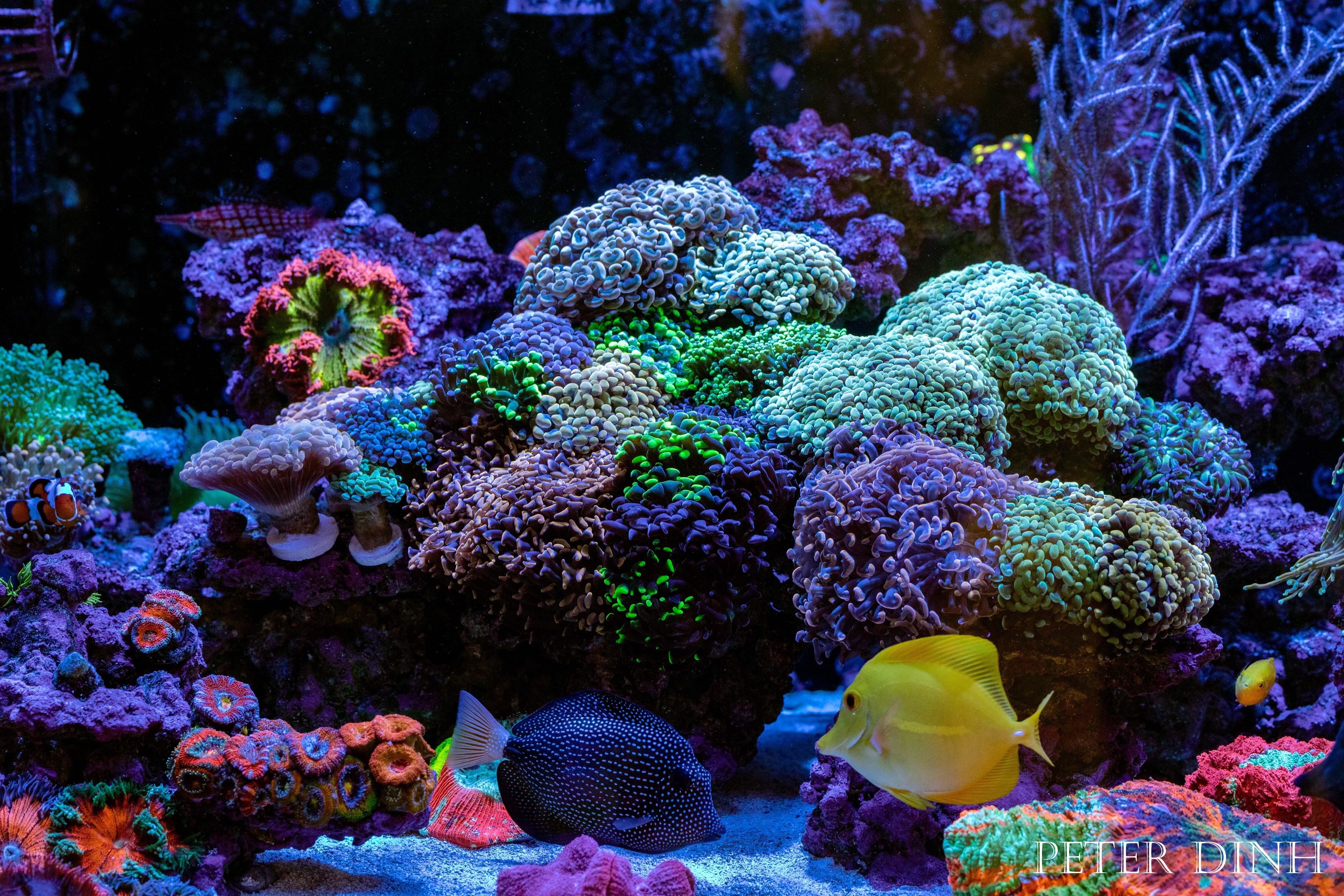This vibrant and colorful underwater image, credited to photographer Peter Dinh, showcases a meticulously crafted aquarium scene that captures the essence of a coral reef. Dominated by a stunning array of neon-like hues, the scene comes alive with glowing purples, greens, pinks, and blues that seem to pop off the screen. The aquarium is teeming with various corals, including red and purple types in the bottom left. Two prominent fish are featured in the foreground: a bright yellow, clownfish-shaped fish and a navy blue speckled fish that resembles a starry night sky. Other aquatic life includes an orange and white clownfish on the left, accompanied by a scattering of purple and pink fish swimming around the coral. The background gradually darkens, adding depth to the scene. The clear image captures intricate details such as the fish’s scales and eyes, creating a lifelike underwater experience.